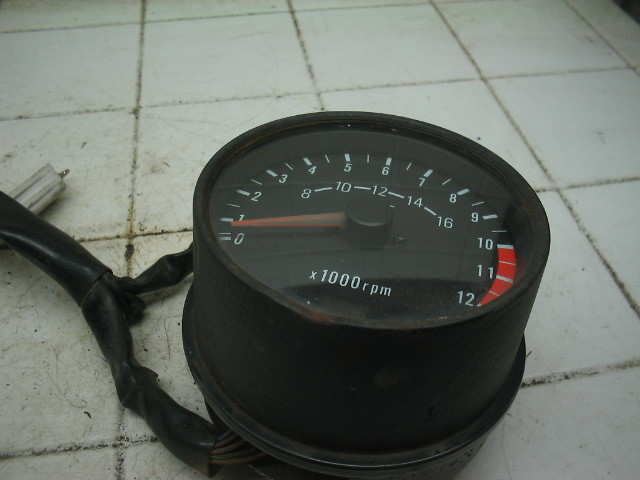This detailed photograph features a black round gauge, specifically designed to measure the revolutions per minute (RPM) of an engine. The gauge's circular face is encased under a protective glass cover and set atop barrel-shaped black sides. This particular gauge appears to have been detached from the engine it originally belonged to, evidenced by the visible cords extending from the left side of the instrument. These cords, originating from two points at the gauge's base, are bound together with black electrical tape, forming a thicker section once combined.

The gauge is placed on a tiled floor, consisting of white square tiles that exhibit numerous scuffs, scrapes, and traces of dirt lodged in the grout lines. The gauge face is predominantly black, featuring a solitary orange dial currently positioned towards the zero mark on the left. Surrounding the dial are incremental dash marks, numerically labeled from zero on the left to 12 on the right. Notable on the gauge face is a highlighted red section spanning from the 10 to the 12 mark, signaling the engine’s maximum safe RPM range.

Beneath the dial, white text indicates the measurements are in thousands of RPMs. Additionally, numbers above the dial increase sequentially from 8 to 16, offering further detail to the gauge's readout.